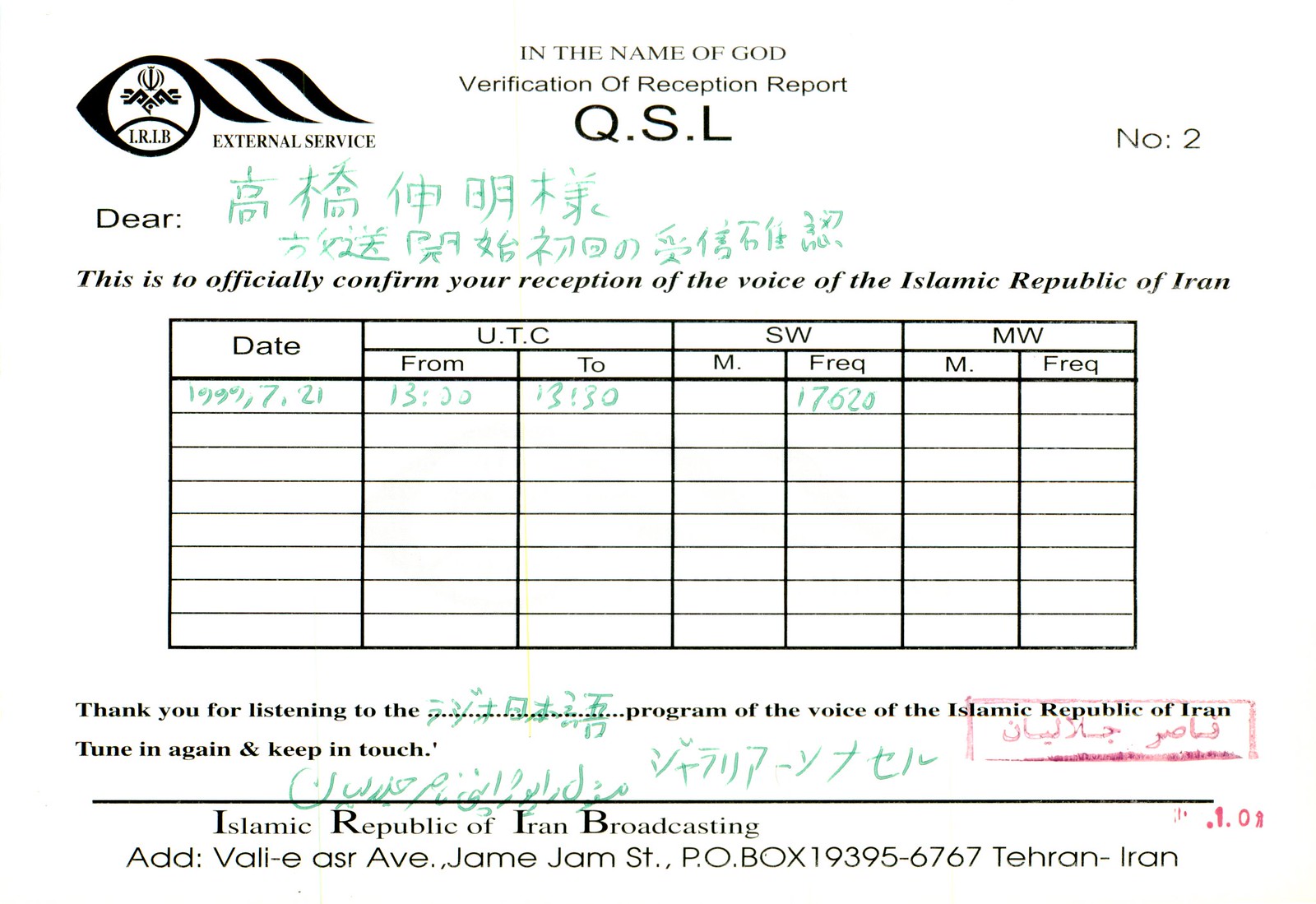The image depicts an official reception report from the Internal Service, confirming the receipt of the Voice of the Islamic Republic of Iran. The report, white with black text, includes green Chinese characters and has a distinct red stamp towards the bottom. At the top center, it begins with “In the name of God” for the verification of the reception report, followed by "QSL." The top left features the IRIB logo, a circle with radiating lines. On the right, it states "NO 2." Central to the image is a table listing DATE, UTC, FROM and TO, SWM and FREQUENCY, MWM and FREQUENCY, detailing the reception dates and timings. The text confirms the reception of the Voice of the Islamic Republic of Iran from Tehran, with a thank you note and a suggestion to "Tune in and keep touch" at the bottom. The document includes signatures and addresses in Tehran, reflecting its official nature.